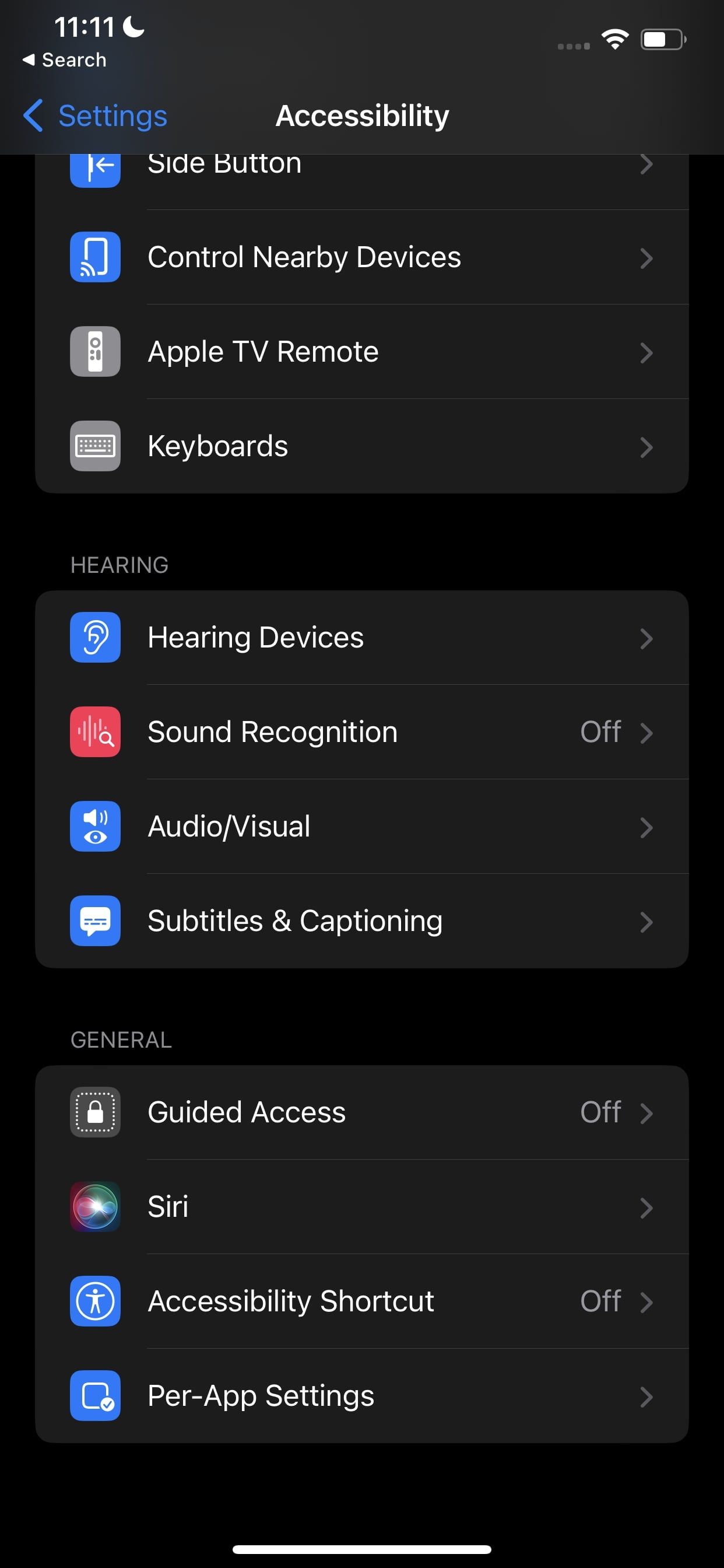This detailed screenshot captures a moment on a person's cell phone's settings menu. The time displayed at the top is 11:11, accompanied by a crescent moon icon, which typically indicates that the device is in "Do Not Disturb" mode. Surrounding the time are the usual status icons: Wi-Fi connectivity and battery life indicator. The screen features a comprehensive list of accessibility options including, but not limited to, "Search," "Settings," "Accessibility," "Side Button," "Control Nearby Devices," "Apple TV Remote," "Keyboards," "Hearing," "Hearing Devices," "Sound Recognition" (currently off), "Audio/Visual," "Subtitles and Captioning," "General," "Guided Access" (off), "Siri," "Accessibility Shortcut" (off), and "Per App Settings." The background of the entire image is a solid black, making the white text stand out clearly. This image is a vertical screenshot with no photographic elements such as people, animals, plants, or any structures, solely depicting the digital interface of the phone's settings.